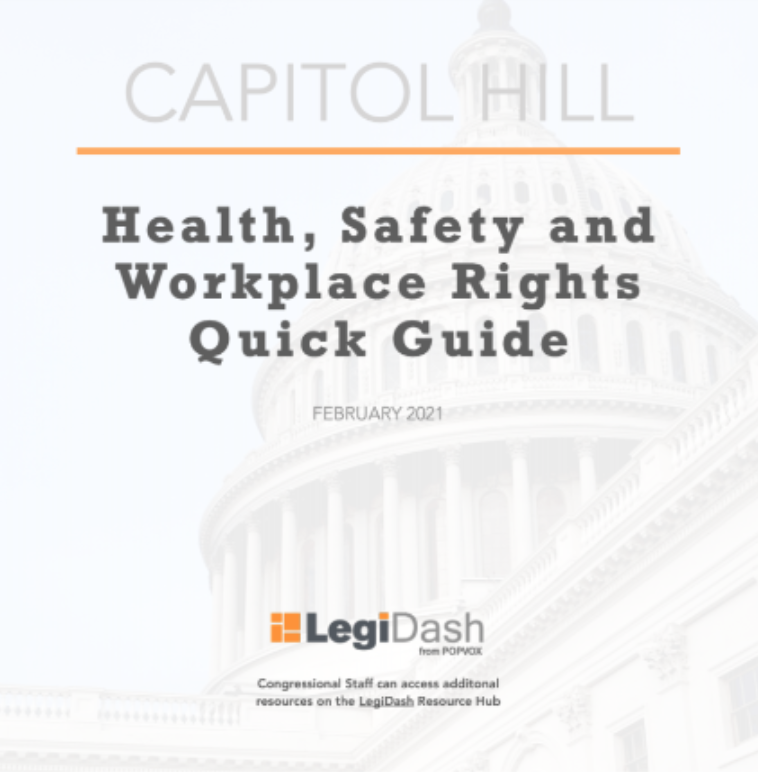This informational brochure, possibly part of a webpage, prominently features a very faint photograph of Capitol Hill with the Capitol building's dome dominating the background. Overlaying the image is a detailed text layout. At the top, it reads "Capitol Hill" in light gray, accompanied by a distinctive orange horizontal line. Below, in bold black text, it states, "Health, Safety, and Workplace Rights Quick Guide," followed by the publication date, "February 2021," in gray. Near the bottom, there's a piece of text that begins with "LEGI-" and further down it notes, "Congressional staff can access additional resources on the LEGI-Resource Hub." This brochure appears to serve as a front-page guide, particularly aimed at informing and reminding Congressional staff about their health, safety, and workplace rights.